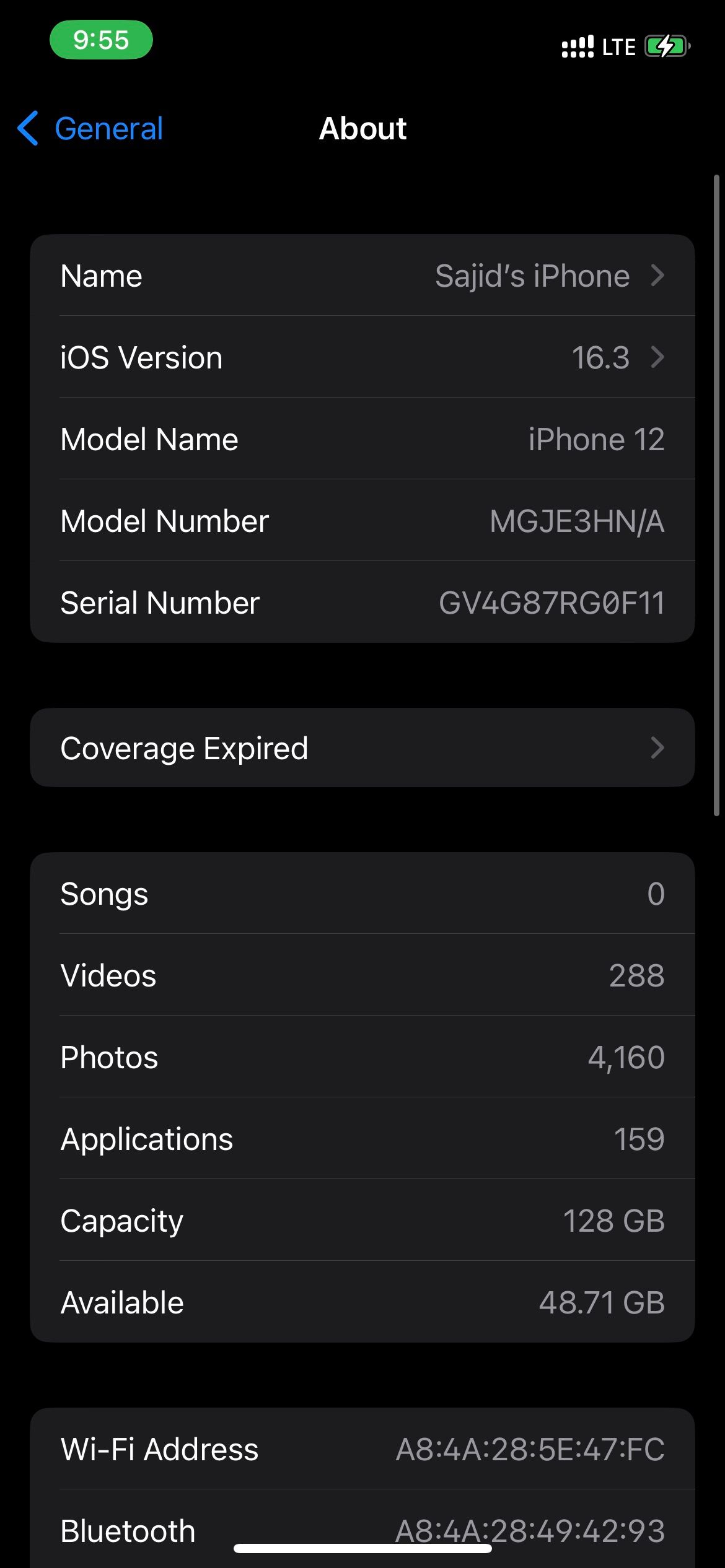The image depicts a cell phone screen showcasing the "About" section within the settings on an iPhone 12. In the top left corner, the screen displays the time "9:55," encased in a small green oval. To the right, standard mobile status indicators are visible, including cellular signal bars, LTE connectivity, and a battery icon, which appears to be charging.

The header of the screen reads "General" in blue, accompanied by a left arrow, and beneath it, the word "About" is prominently displayed in white. The detailed device information listed includes:

- **Name**: SAJID’s iPhone
- **iOS Version**: 16.3
- **Model Name**: iPhone 12
- **Model Number**: MGJE3HN/A
- **Serial Number**: GB4G87RG0F11
- **Coverage**: Expired
- **Songs**: 0
- **Videos**: 288
- **Photos**: 4160
- **Applications**: 159
- **Capacity**: 128 GB
- **Available Space**: 48.71 GB

Additional network data provided includes:

- **Wi-Fi Address**: A8:4A:28:5E:47:FC
- **Bluetooth Address**: A8:4A:28:49:42:93

The overall text is rendered in white or gray against a black background, providing a clear and high-contrast layout for easy readability. Running across the bottom of the screen is a thin white line, demarcating the end of the detailed information.